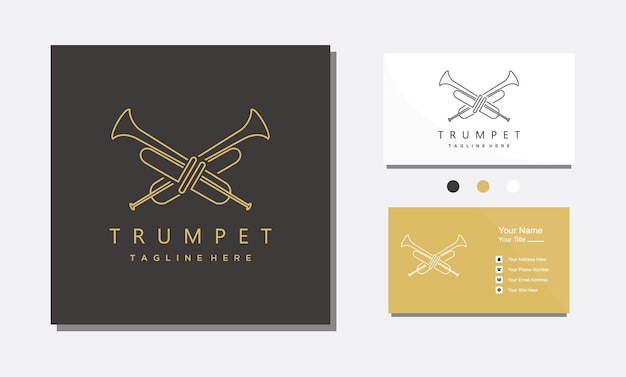The image showcases a promotional package prominently featuring a unified branding concept centered around the word "TRUMPET." On the left side of the image, there is a sleek, geometric line drawing of two intersecting trumpets in an X shape, rendered in a gold shade against a black background. The word "TRUMPET" is displayed boldly in all caps, larger than the smaller tagline "tagline here," both in the same gold color. 

To the right, two business cards are displayed side by side, representing the front and back designs. The top card has a white background with the same trumpet line drawing in black, accompanied by the text "TRUMPET tagline here" and three dots in black, yellow ochre, and white. The bottom card features a yellow ochre background with the trumpets and text "Your Name Here" followed by four vertical points, indicating placeholders for additional information. The overall design is minimal yet sophisticated, emphasizing consistent use of color and geometric elements across the materials.